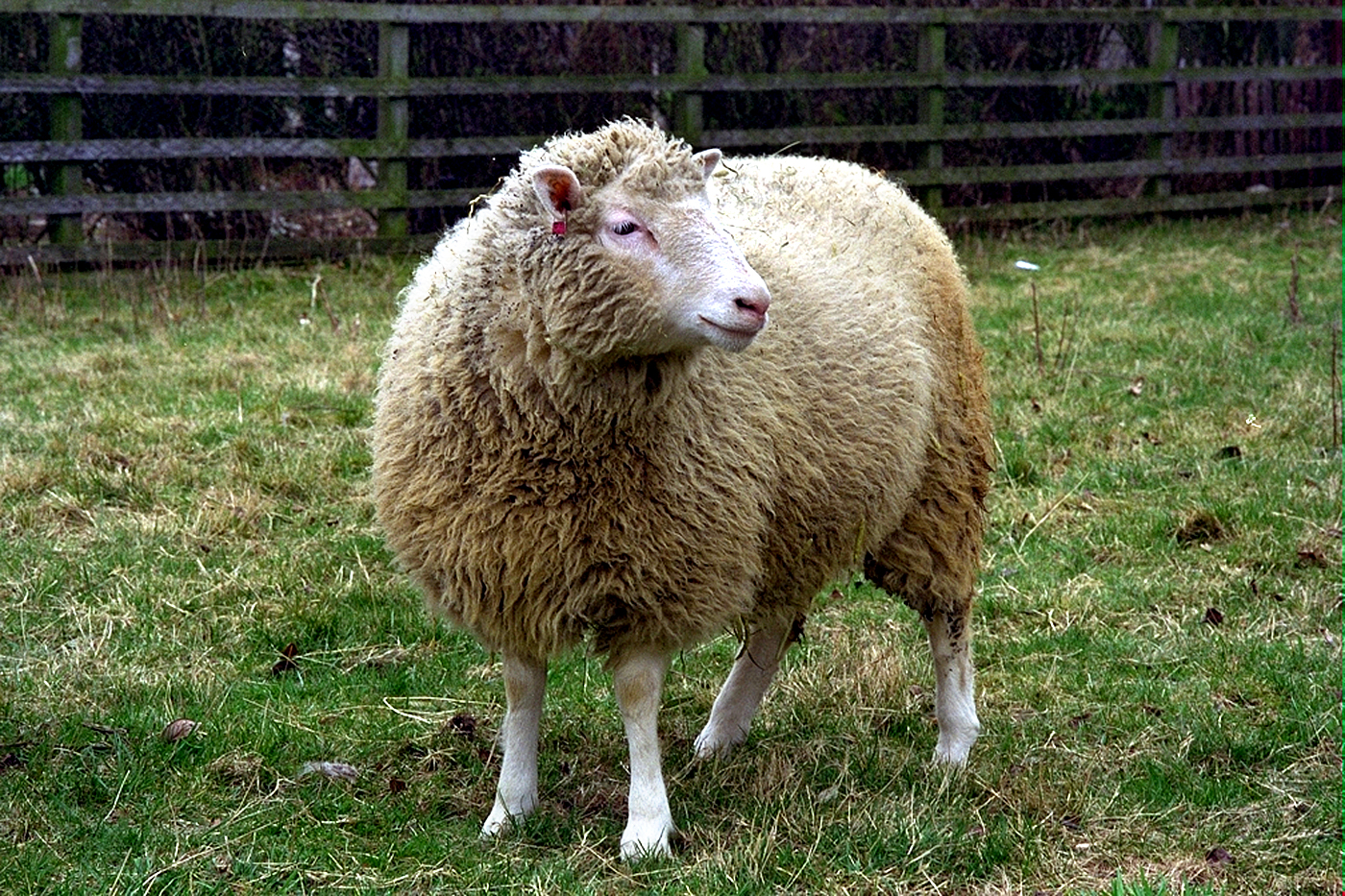This photograph captures a large, woolly sheep standing in the center of a grassy field, which appears to have some straw strewn about. The sheep is the main focal point, with its body facing left and its head turned right, giving the impression it is looking at something off-camera. Its wool transitions from a light brown at the top to an almost white towards the legs, though it has a dirty, brown-tinged appearance. The sheep's face and legs are white, and it sports a red tag in its ear. The background features a wooden slatted fence running the full length of the image, parallel to a wire fence. This fence, combined with the grassy area, suggests the sheep is in a pen. The sheep looks remarkably fluffy and even seems to have a slight smile on its face, adding to its endearing presence in the photograph.